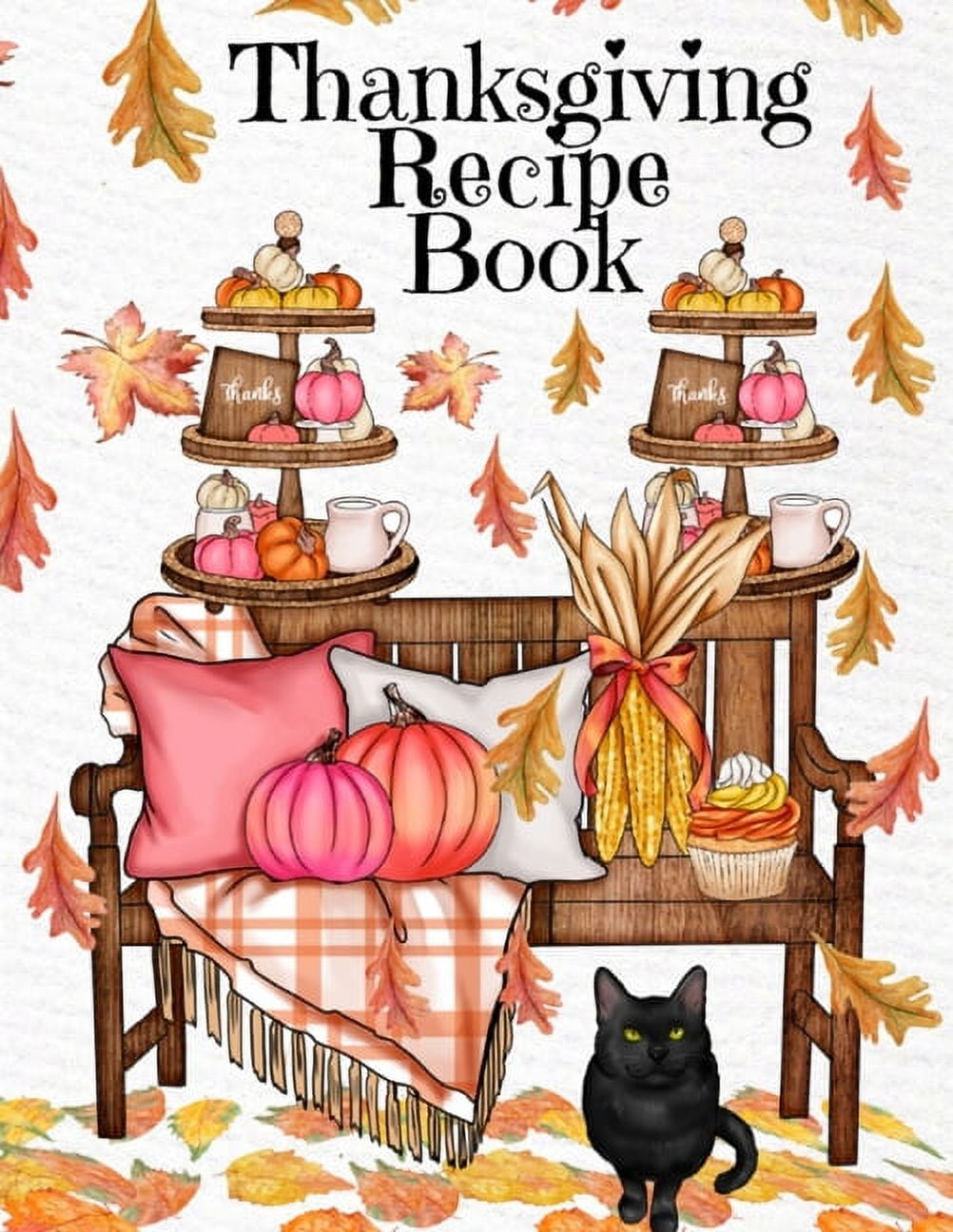The cover of the book titled "Thanksgiving Recipe Book" features a charming, illustrated design with a white background adorned by brown, autumn leaves. In the center, a wooden bench holds an array of Thanksgiving-themed decorations. To the left, a cloth with yellowish-orange stripes, throw pillows, and pumpkins are arranged on the bench. On the right, a bundle of corn and a cupcake add to the cozy aesthetic. Multiple racks of food flank the bench, along with a coffee cup and small pumpkins. Below the bench, a black cat with green eyes, slightly leaning forward, looks directly at the viewer. This delightful illustration conveys a warm, festive atmosphere perfect for Thanksgiving.